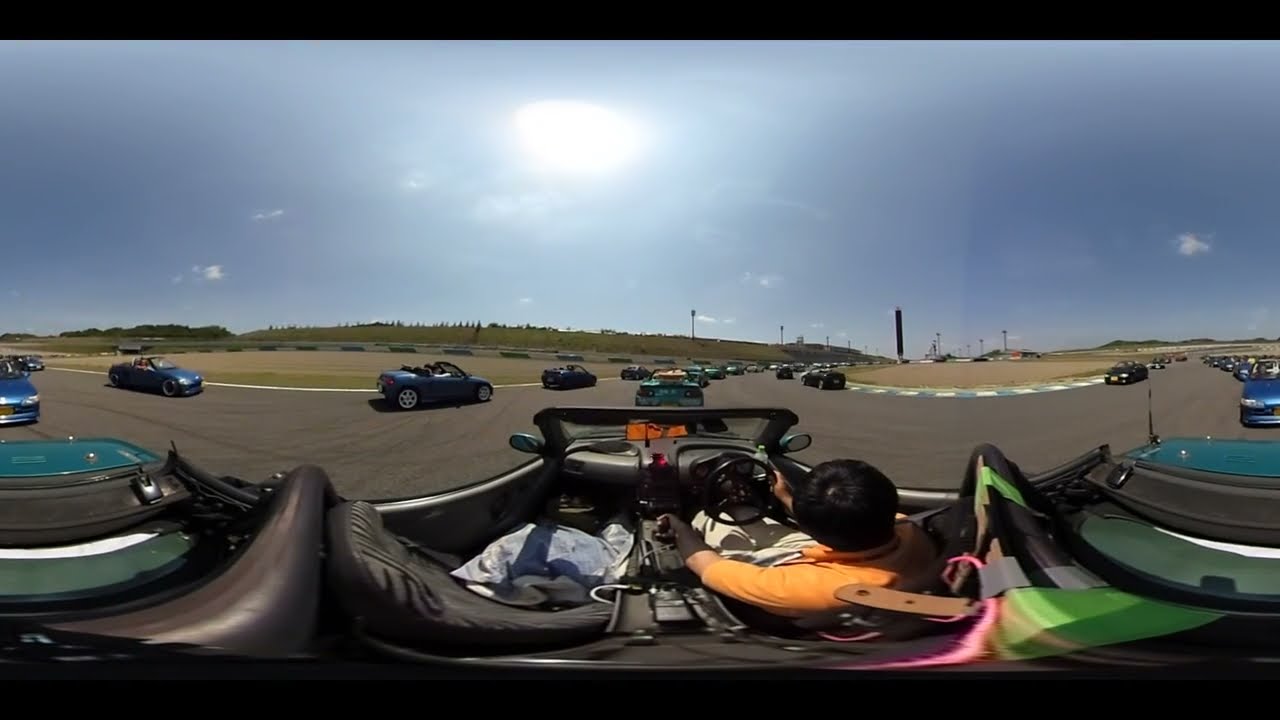The image is a detailed, panoramic 360-degree shot, capturing the dynamic scene of a go-kart race on a sunny day with a clear blue sky. The foreground reveals the interior of a sports car, showcasing black seats and a rectangular black frame in the front with tiny mirrors on either side. A man with black hair, wearing an orange shirt and brown trousers, is in the driver's seat, one hand gripping the steering wheel and the other on the gear stick. Beside him, the left side seat is unoccupied.

The race track curves and bends throughout the image, with a gray surface and blue and white squares marking the sides. Numerous blue convertible go-karts fill the track, approximately fifteen or more, navigating the curved path. At the front of the image, a grayish structure adorned with vertical lines and a turquoise metal cap on either side is visible. In the backdrop, there's a bright white sun in a clear blue sky, emphasizing the vivid, sunny setting of the race. The overall atmosphere exudes excitement and motion, encapsulated within the high-energy race.